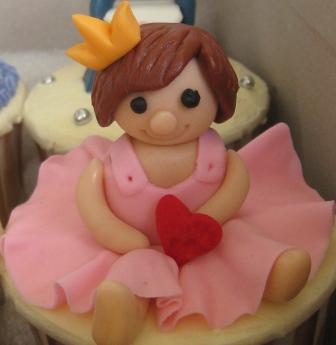The image depicts a detailed, fondant cupcake topper shaped like a cute little girl with a chubby body. She is seated on a white disc, surrounded by a flowing, rippled pink skirt resembling a tutu. The little girl's feet are visible at the front, and her arms are crossed at her waist, holding a small red heart in her left hand. She wears a pink dress with little straps, and her short brown hair, styled with bangs swaying to one side, is adorned with a yellow bow on the top left edge. Her face features black eyes, a round button nose, and a drawn-on smile. Perched on her head is a tiny three-pointed crown. Behind the figurine, there's another cupcake decorated with silver nonpareils and blue piped frosting, emphasizing that the entire scene is part of a larger confection made from edible materials like fondant, marzipan, and frosting.